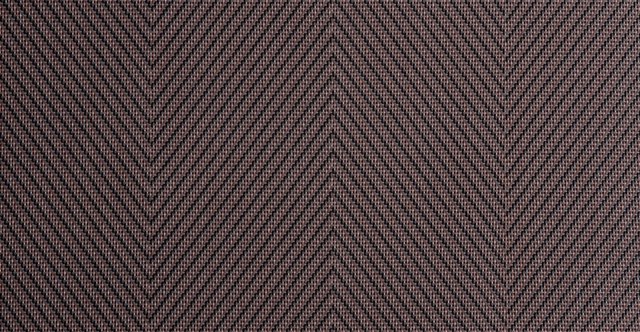This horizontal rectangular image features an intricately patterned fabric swatch. The fabric is divided into four sections from left to right. In the first section starting at the bottom left corner, there are dark stripes that diagonally traverse from the upper left to the lower right. These stripes gradually become smaller as they ascend to the section's midpoint, beyond which they continue but diminish in size. The stripes form distinct, connected V shapes at the boundaries between sections. Each subsequent section mirrors this pattern, creating an alternating sequence of dark upward and downward V-shaped lines.

In the second section, these V's continue to form at the point where the first section ends, riding up and to the right, and then interconnecting with the third section where the V's reverse direction, heading down and to the left. This interconnection continues into the fourth section, maintaining the repetitive V-pattern symmetry. The fabric has a background of lighter purple interspersed with some subtle dashes that add texture to the material.

The overall coloration includes hues of blue-gray with touches of pink and purple, set against dark V-shaped markings that appear almost black or dark brown. The material is tightly woven, resembling fabric like gabardine, and features rows of these geometric V patterns interchanging against a textured backdrop, emphasizing the fabric's rich, structured weave.